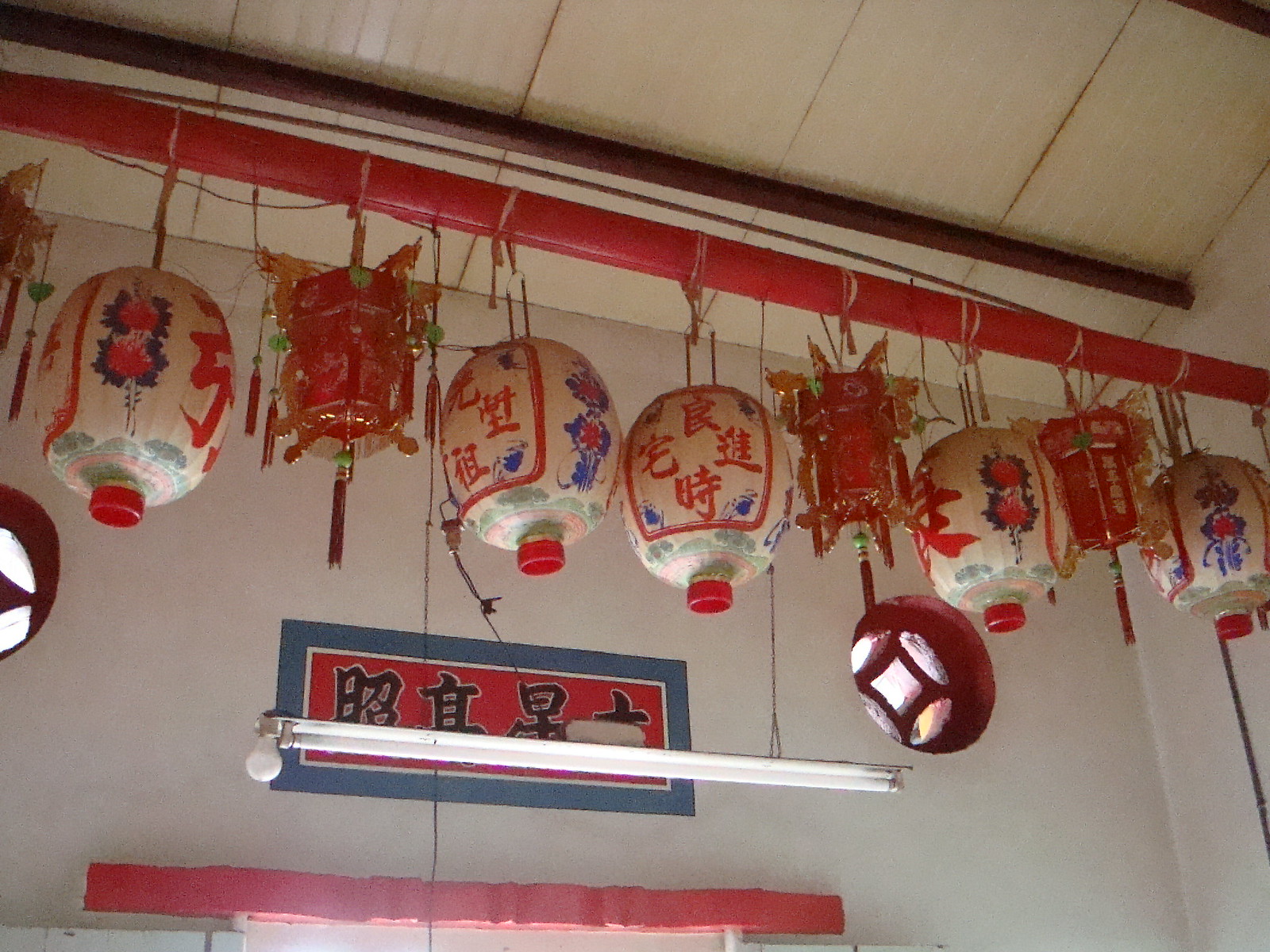This photograph showcases an indoor scene with several Chinese lanterns hanging from a bright red cylindrical beam near the ceiling. The setting appears to be a room with white and off-white walls and ceiling, which is angled and features additional details like a red pipe, possibly part of the structural or decorative elements. Fluorescent lights are also visible, suspended from the ceiling. 

The lanterns are of two distinct designs. There are five oval-shaped white lanterns embellished with large red text and blue and red floral patterns. They have a green and orange ring on the underside, with a small red circle protruding at the very bottom. The second design consists of more ornate, hexagonal red lanterns adorned with faint gold patterns and multiple gold prongs sticking out, from which long red tassels hang, featuring a green disc in the middle. 

Arranged in a pattern, these lanterns collectively add up to eight fully visible ones, with a ninth lantern partially cut off at the far left edge of the image. The sequence begins with an oval white lantern, followed by an ornate red one, and continues alternating except for the cut-off ornate lantern at the beginning. Also visible in the background is a banner with a blue border displaying Chinese characters in black on a red background, partially obscured by the lanterns. The photograph has a slightly grainy, old-fashioned quality, suggesting it may have some age to it. Two small, high windows with red diamond-pane details can also be seen, contributing to the room's authentic and traditional Chinese aesthetic.